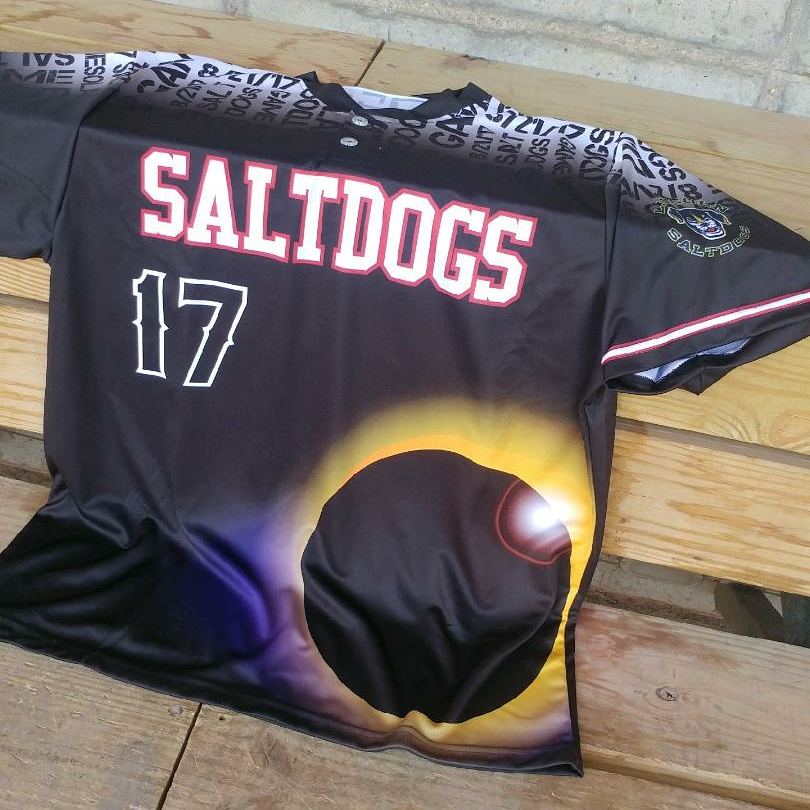A highly detailed photograph depicts an indoor setting featuring a Salt Dogs sports jersey placed on a wooden bench. The jersey, primarily black, prominently displays the text "Salt Dogs" in white with red borders across the chest. Below the team name, the number 17 stands out in black with white outlines. The most striking feature of this jersey is the bottom right corner, which showcases an intricate graphic of a black asteroid with a yellow and purple tail moving diagonally downward towards a formation of gray rocks, resembling an eclipse at the diamond ring stage. The top part of the jersey has some white markings with numbers and letters, though they are somewhat illegible. The left sleeve bears the Salt Dogs' team logo, which includes an image of a dog. The jersey rests on a bench constructed from a couple of wooden planks, light gray in the foreground and lighter brown above. The backdrop indicates an unfinished concrete wall, enhancing the rustic, indoor atmosphere of the image. The jersey appears to be made from high-quality, advanced material, indicating it's a high-tech sports attire.